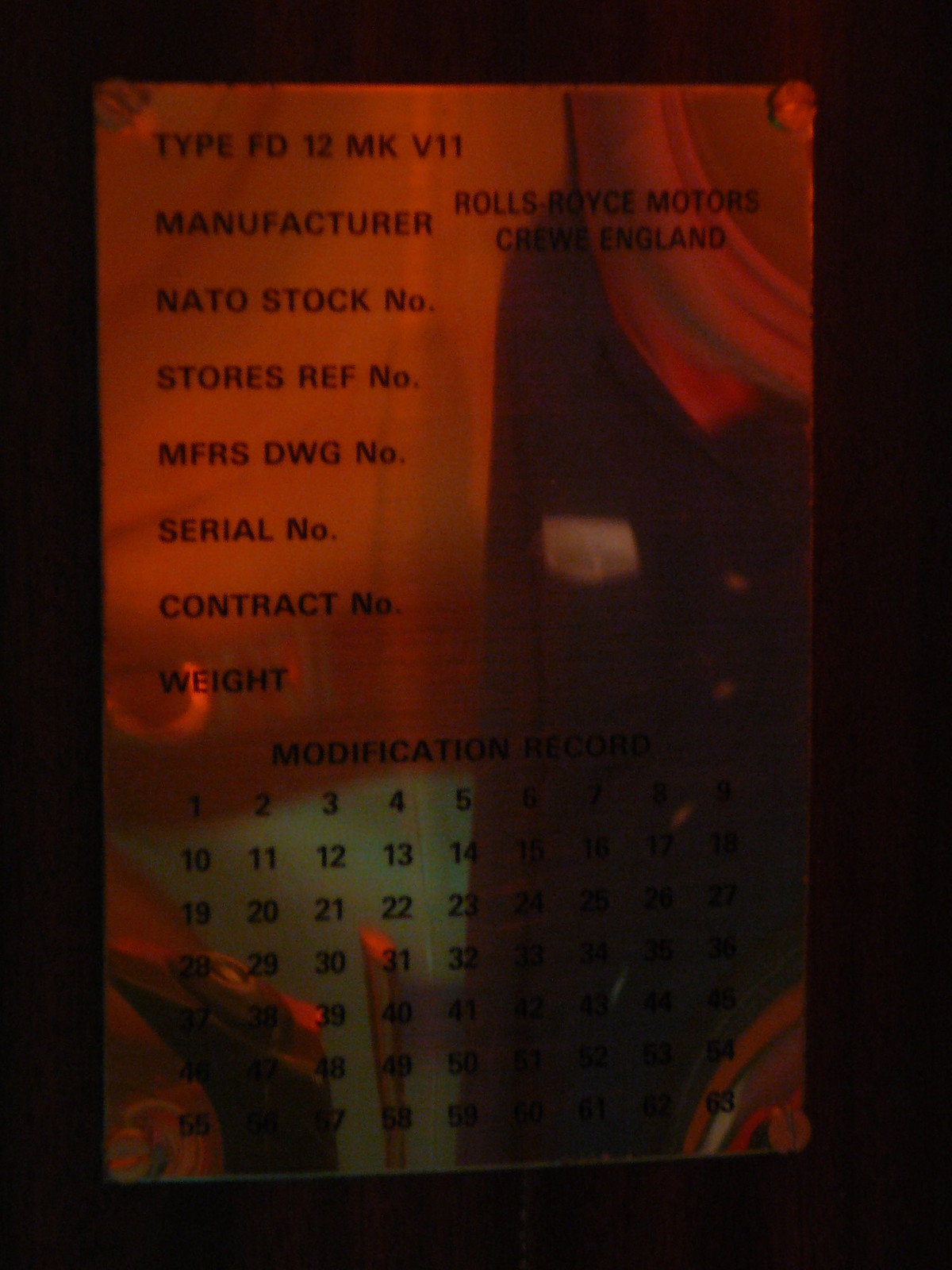The image depicts a close-up view of a glossy metallic sign, positioned centrally against a dark backdrop. The setting is dimly lit, adding to the enigma of the scene. The sign itself bears significant detail, suggesting it may be related to automotive or mechanical use, possibly from a Rolls-Royce vehicle.

At the top of the sign, text in black reads: "Type FD-12 MKV-11, Manufacturer Rolls-Royce Motors, England, NATO stock number, Stores Ref Number, MFR/SDWG Number, Serial Number, Contract Number, Weight, Modification Record." The lower portion is dominated by a calendar-like section with numbers running from 1 to 63, hinting at some sort of modification or maintenance log. This part of the sign is infused with a greenish tint, contrasting subtly with the predominantly black and gold color palette.

Notably, the sign is detailed with black, gold, yellow, and a hint of light blue, providing a touch of color amidst the otherwise shadowy environment. The overall clarity of the image is decent despite the dim setting, allowing the viewer to distinguish the various imprints and the somewhat blurred background, which vaguely resembles auto parts. The image is a portrait orientation photograph with a strong focus on mechanical realism and representational details.